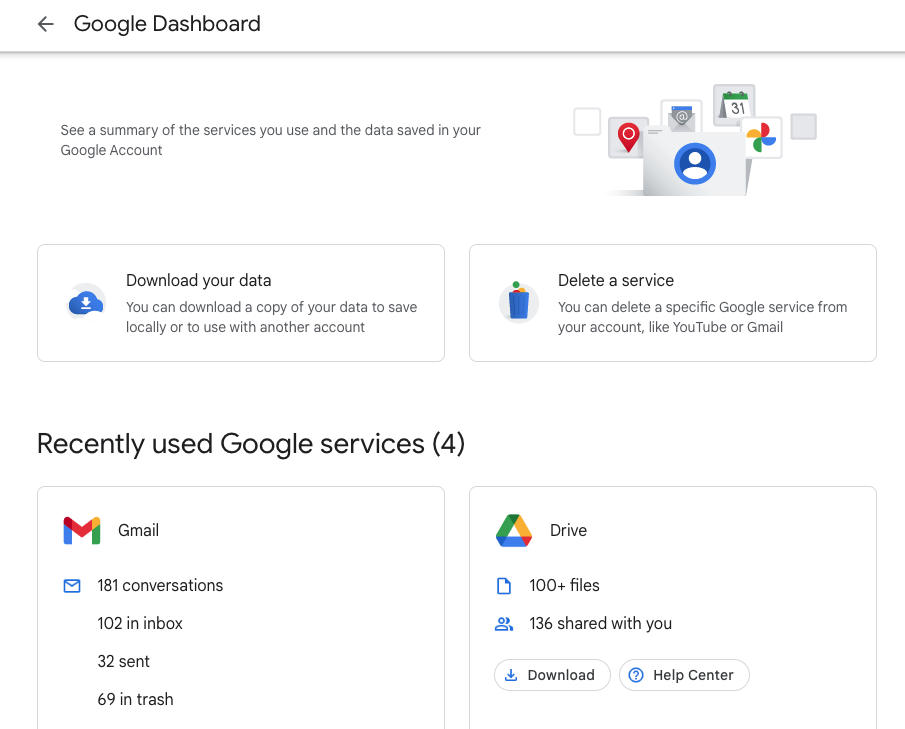The image showcases a detailed screenshot of the Google Dashboard. The primary background color of the dashboard is white, with black text prominently displayed at the top that reads "Google Dashboard," accompanied by an arrow. A gray bar segregates the dashboard heading from the main content area. Below this bar, there's an informative sentence stating: "See a summary of the services you use and the data saved in your Google account."

The page is populated with various sections and boxes, each featuring different Google services and their respective icons. These icons include a calendar icon, the multicolored Google symbol resembling a fan (yellow, red, green, and blue), a blue circular profile icon with a white silhouette, an email icon, and a red pin icon symbolizing location.

One prominent square box on the page is labeled "Download your data." It provides users the option to download a copy of their data for local use or to transfer to another account. This section features a cloud icon with a download button.

Another section titled "Delete a service" offers users the option to remove specific Google services from their account, such as YouTube or Gmail. This is indicated by a circle icon with a trash can graphic.

The "Recently used Google services" section provides a summary of recent activity across various Google services, denoted by 'four' in brackets. Detailed statistics are provided for Gmail, which shows 181 conversations—with 102 in the inbox, 32 sent, and 69 in the trash—accompanied by the Gmail logo. Similarly, the Google Drive icon is present, indicating recent usage.

This detailed screenshot offers a comprehensive view of the user's interactions and data management options within the Google Dashboard.